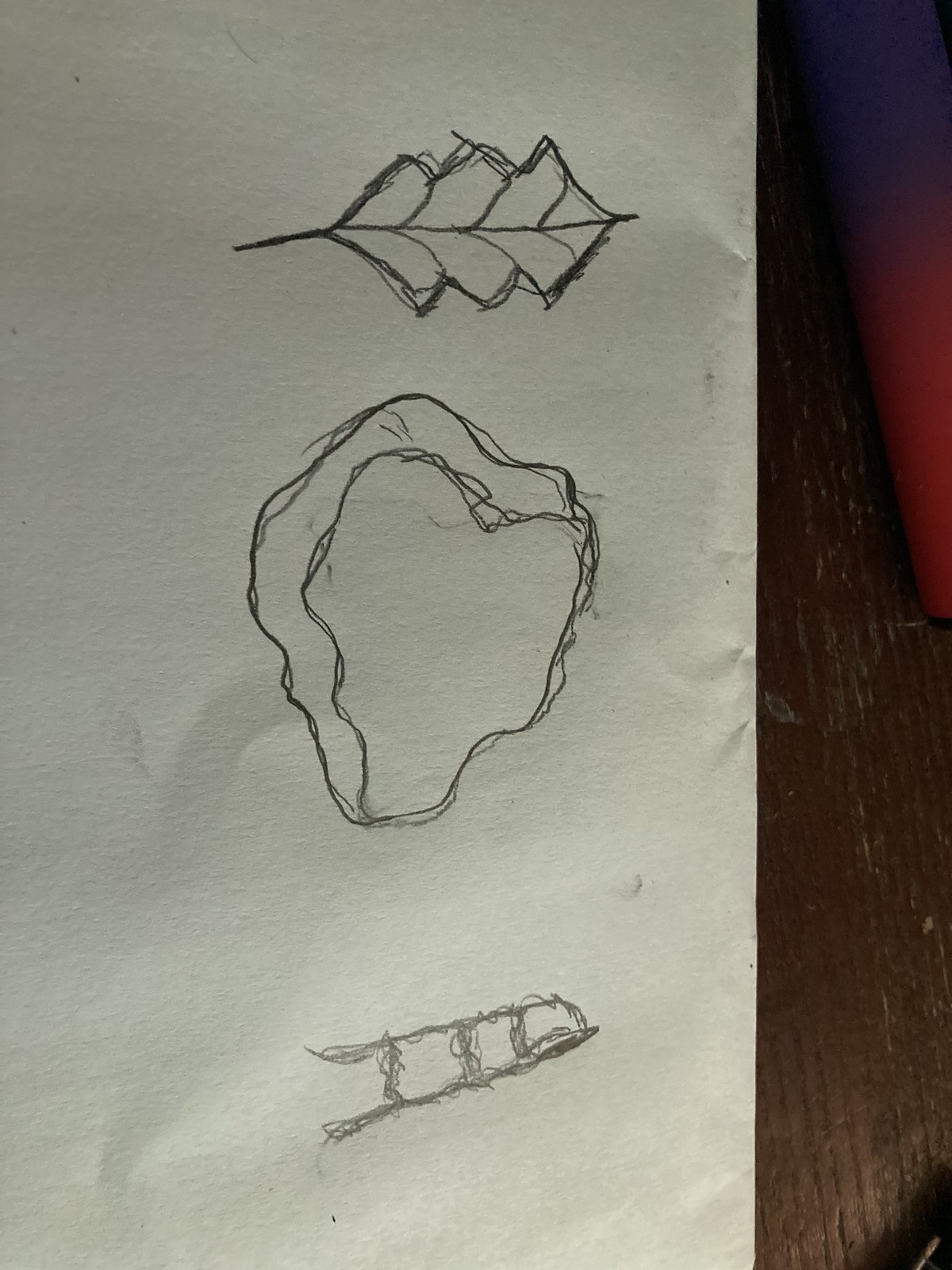On a wooden table lies a piece of paper featuring three distinct pencil etchings. The top etching portrays three heart-shaped figures, although the heart at the very top resembles a square more than a heart, each with a line running through them. Below this, the second etching consists of two main squiggly lines with smaller squiggly lines surrounding them, forming a shape that resembles a jagged circle. The final etching at the bottom of the page represents a ladder-like shape, with short, squiggly lines positioned between two thicker, yet also squiggly, lines.